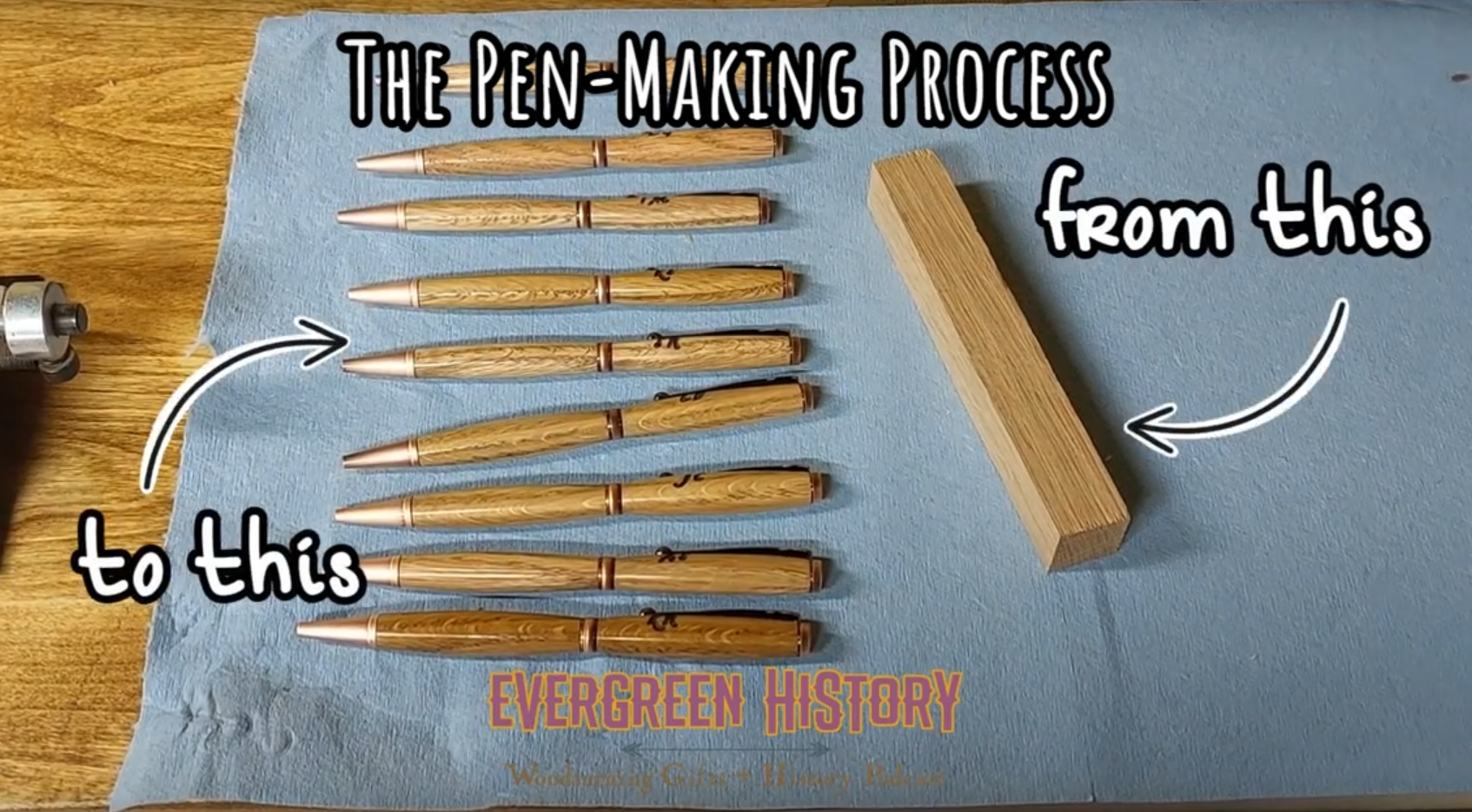The image titled "The Pen-Making Process" illustrates the transformation of a block of wood into handcrafted wooden pens. On a blue piece of cloth or paper resting on a wooden table, the scene features a series of eight pens made primarily from wood, each with a copper end and a metal clip, arranged neatly in a row. An overlay of white text reads "The Pen-Making Process," with an arrow starting from a labeled block of wood on the upper left, arcing downward to the right labeled "from this," and another arrow arching upward to the pens labeled "to this." Below the row of pens, the words "Evergreen History" are written in orange. The silver end of an unspecified tool, possibly a lathe, suggests the woodworking method to create the pens. Additional text includes "Woodworking Gifts" and two other indistinguishable words.